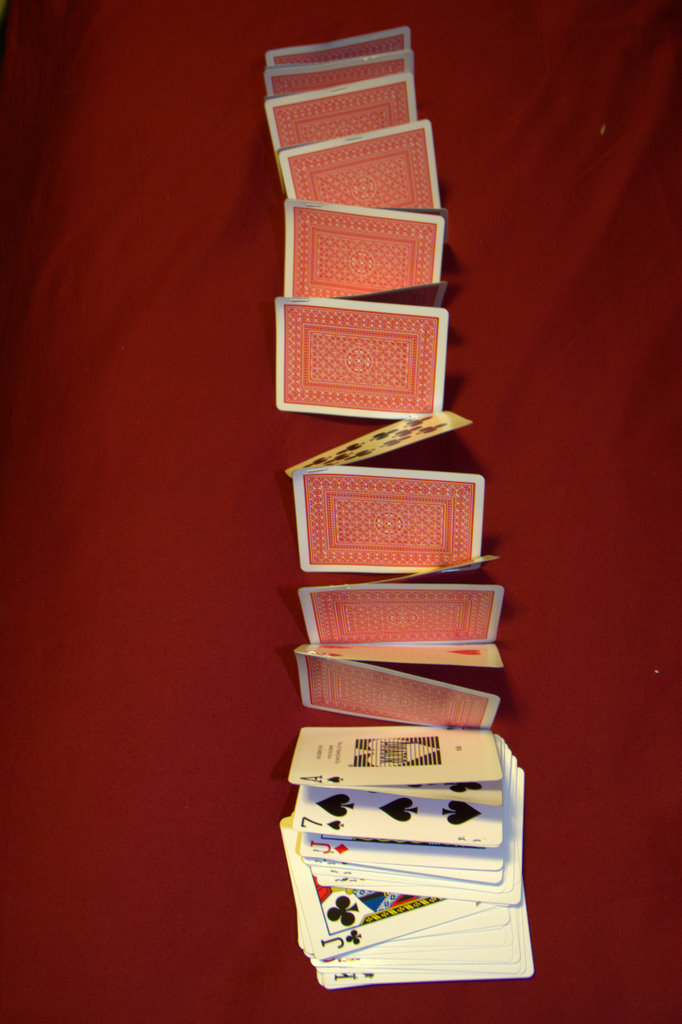The image features a vibrant red background with what appears to be a scattered deck of cards either carelessly dropped or meticulously arranged. The cards, adorned with a generic red back design, seem to cascade from the top to the bottom of the image. Towards the bottom, the majority of the cards are face up, revealing their traditional designs. Approximately 15 to 20 cards are suspended in mid-air, emphasizing their disordered state. Some cards are positioned at various angles, showing a mix of card faces and backs. The cards appear thoroughly shuffled, indicating no particular order, characteristic of a standard deck found in common card-playing venues.